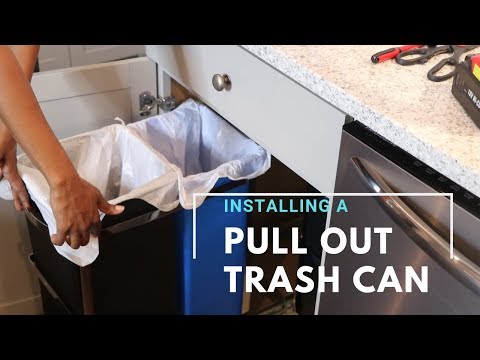The image, titled "Installing a Pull-Out Trash Can," depicts a kitchen setting where a pair of pull-out trash cans are being showcased. The trash cans, one black with a white liner and another blue with a white liner, are mounted in a pull-out holder situated beneath a cabinet. The pull-out mechanism serves both a trash bin and a recycle bin. A person with dark skin is interacting with these bins, either pulling them out or putting them back in, with their hands and arms visible on the left side of the image. Above this setup is a white drawer with a round, silver handle, and to the right of the cabinets is a stainless steel dishwasher. The countertop is white with black speckles, holding various tools such as screwdrivers and scissors. Overlaid text on the image reads "Installing a Pull-Out Trash Can." This image could serve as an advertisement or a still from a how-to video, showcasing the practical and organized nature of a pull-out trash can system in a kitchen setting.